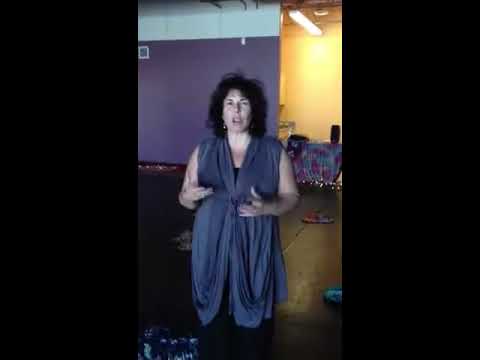The image depicts a white woman with shoulder-length, dark brown hair that has a slight curl to it. She stands facing the camera with her arms raised at her sides and hands extended outward, seemingly in the middle of speaking or explaining something. Her mouth is open, adding to the impression that she is talking. She is dressed in a soft dark purple dress or a long, baggy shirt that ties at the waist, extending down to about her knees. The woman stands on a dark brown or black floor. The background wall behind her features a combination of soft purple and white colors, transitioning approximately two feet from the top. There are also hints of aqua and yellow tones. Surrounding the vertical frame of the image are solid black borders on both sides, about an inch thick. Additionally, there appears to be a ceiling fan visible above her.